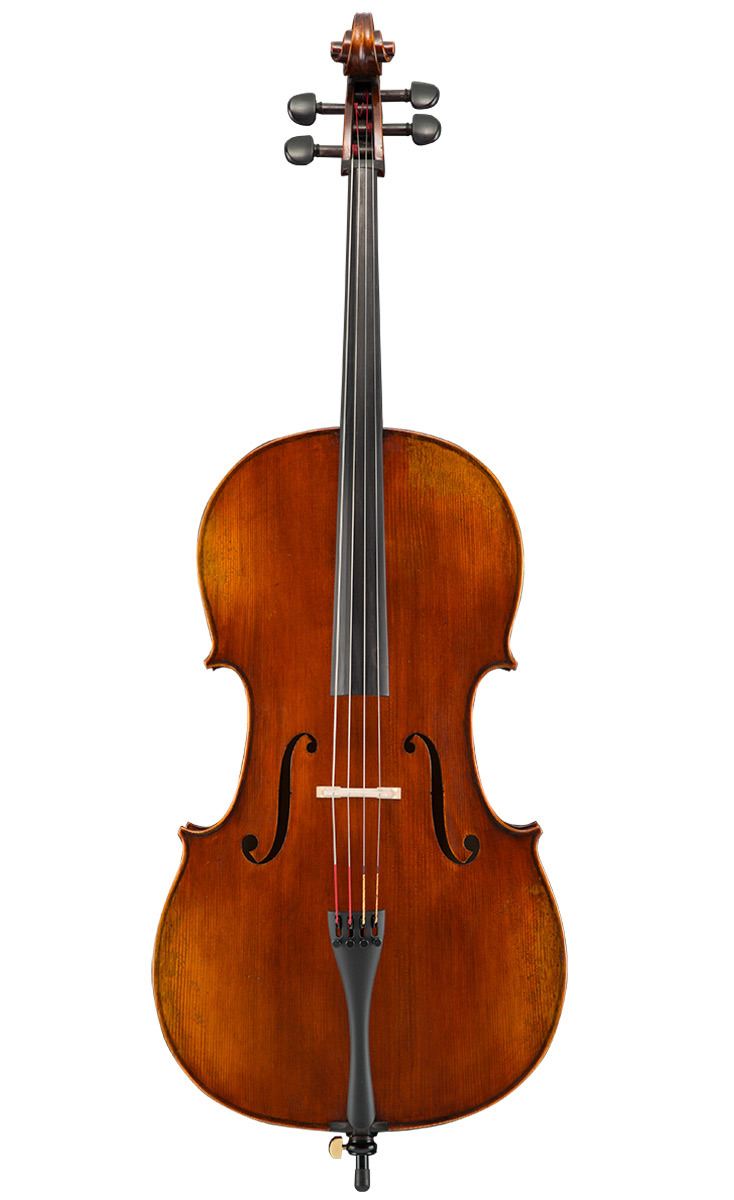This is an image of a four-stringed wooden violin, standing upright against a completely solid white background, making it look like a product photo. The violin's body is crafted from a cherry wood that gives it a rich brownish-orange hue with touches of gold. The violin features distinctive 'f' holes on either side of its center, characteristic of stringed instruments. The instrument's neck and the tuning pegs, which tighten the strings, are black, likely made of plastic. The violin is in excellent condition, appearing photorealistic with no signs of wear or decoration such as stickers. There is no bow visible in the image, and no additional accessories or background elements, emphasizing the elegant simplicity of the instrument itself.